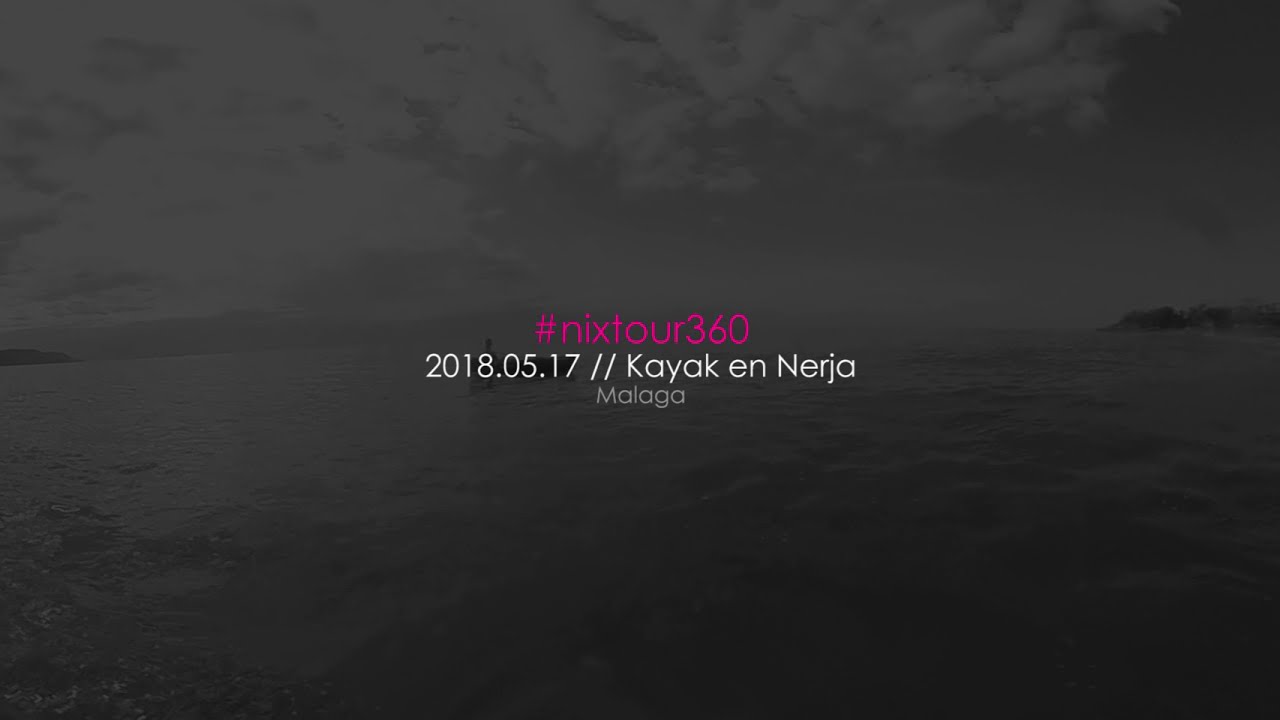The image is a rectangular, intentionally darkened or filtered, black and white photograph depicting a body of water, framed as if taken from the water level. The water appears calm but not entirely smooth, suggesting some movement. The background sky is partly cloudy, with the right half clearer and the left half filled with wispy clouds. Along the horizon, snippets of land are visible on both the left and right sides, indicating a cove or shoreline area protruding into the scene.

Dominating the center of the image is a bold, hot pink text overlay of the hashtag "#NYXTOUR360". Directly below in white text is the date "2018.05.17", followed by the phrase "Kayak en Nerja", and further beneath it, the word "Malaga" in a smaller white font. Despite the text superimposed over it, there is a faint outline of what appears to be a kayak floating in the water. This image, likely an advertisement, suggests an event or service related to kayaking in Nerja, Malaga.